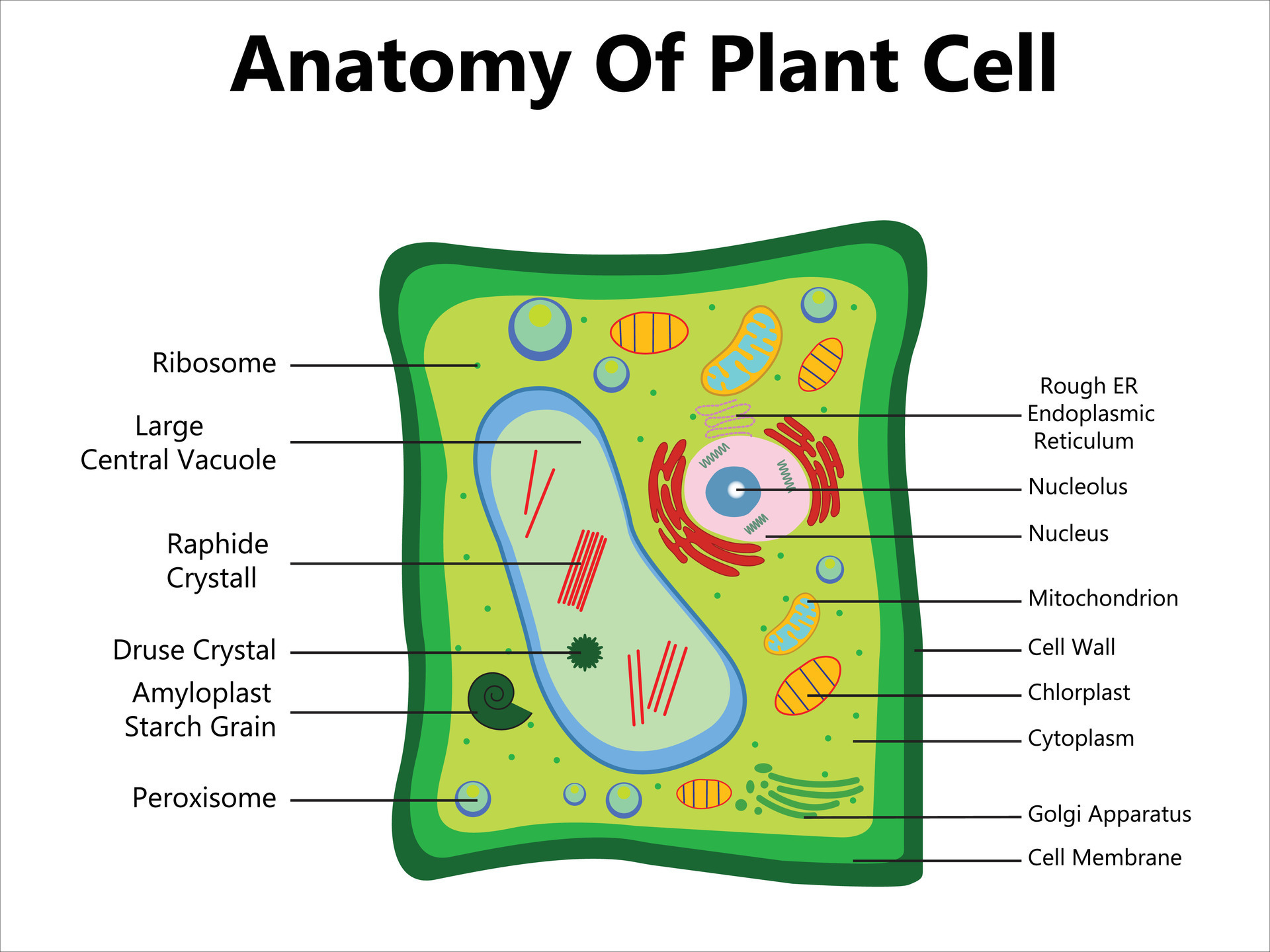The diagram titled "Anatomy of a Plant Cell" showcases an illustrated plant cell against a white background. The central feature is a large, horizontally oriented rectangle with a dark green outer border and a lighter green inner border, depicting the cell wall and cell membrane, respectively. The inner area, illustrated in a lighter green, represents the cytoplasm and contains various labeled organelles.

Prominent organelles include:
- The **nucleus**, depicted as a large, pink circular structure with blue inner detail and strings of red surrounding it, along with a labeled nucleolus.
- **Chloroplasts**, shown as oval structures with vertical black lines.
- The **mitochondria**, yellow bean-shaped forms with blue internal "rivers".
- The **rough endoplasmic reticulum (Rough ER)**, depicted as thin brown strings.
- The **Golgi apparatus**, illustrated at the bottom left with a curved, stacked appearance.
- The **amyloplast (starch grain)**, represented as a green, shell-like structure.
- The **large central vacuole**, occupying most of the cell's space, with blue walls and containing red raphid crystals and star-shaped druse crystals.

Throughout the cell, smaller organelles and components such as ribosomes and peroxisomes are labeled and linked with lines. The diagram provides a comprehensive visual guide to the plant cell's anatomy, utilizing a visually accessible cartoon drawing style.